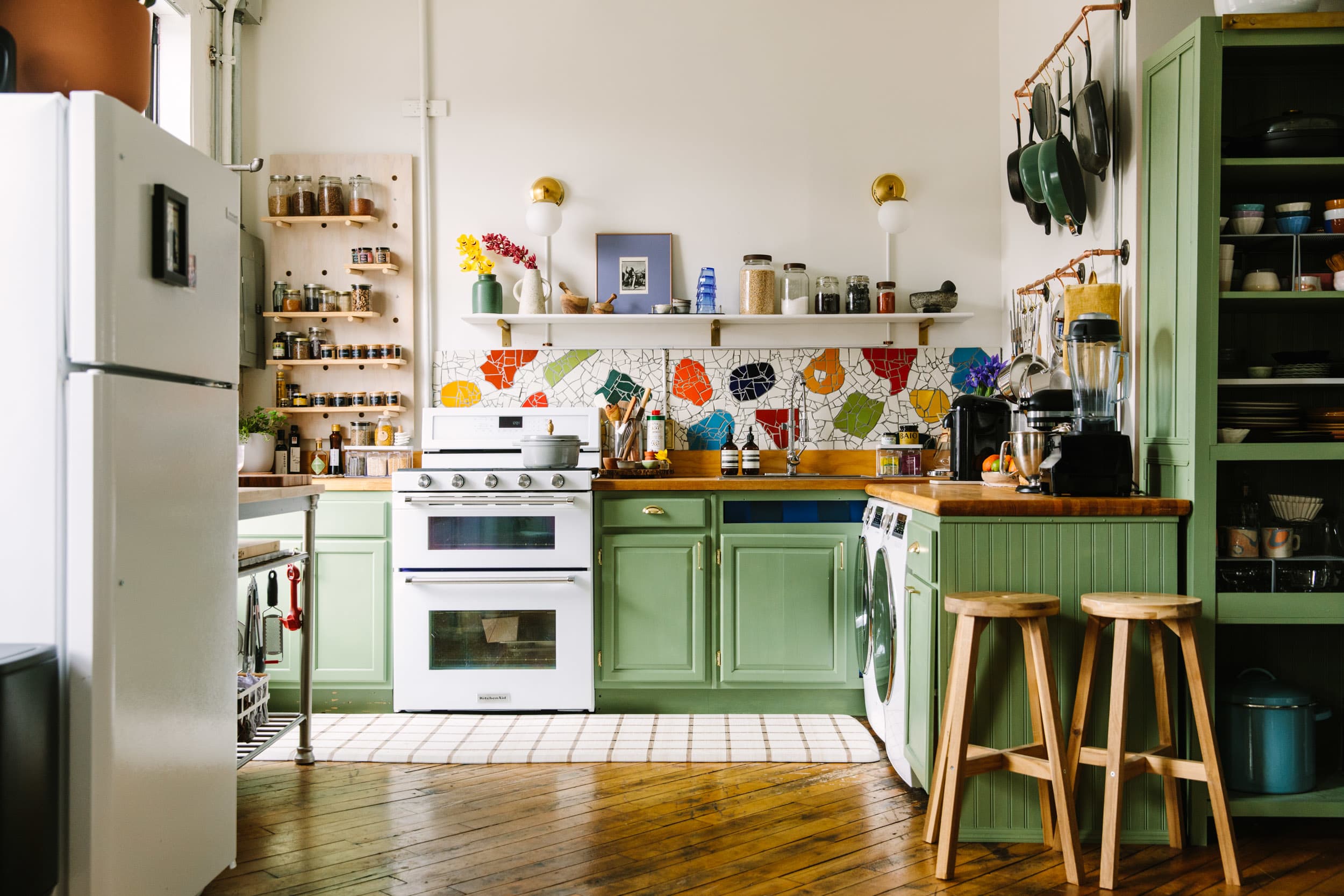This detailed image captures a cozy, well-used kitchen with vintage charm. Predominantly featuring a compact space, the kitchen boasts an old-style white stove equipped with a broiler on top and an oven below. The surrounding cabinetry is painted a medium sea green, providing a vibrant contrast to the white appliances. Notably, there is a white refrigerator with a top freezer on the left side of the room, completing the vintage feel.

The countertop, constructed from light brown wood and designed in an L-shape along the right and far walls, is adorned with a variety of appliances including a coffee maker, a blender, and an espresso machine nestled in the far-right corner. Further enhancing the functionality of the space are small floating shelves on the walls, filled with an array of spices and seasonings. 

Above the countertop, a white shelf spans the area, dotted with decorative items like jars and glasses, and flanked by two sconces. Directly in line with the shelf is a backsplash of white tiles interspersed with colorful mosaic clusters of orange, green, yellow, dark green, black, blue, and purple, adding a playful touch to the room.

The floor, made of shiny wood tiles arranged in diagonal slats, features a mix of medium and dark grains, contributing to the kitchen's warm and inviting ambiance. Two small wooden bar stools with matching legs are positioned at the end of the counter, providing a cozy seating area.

Completing the layout, the kitchen also includes a washer and dryer subtly integrated into one of the counter cabinets. The light, amber-toned wooden flooring, combined with the thoughtful blend of décor and practical elements, underscores the quaint, functional charm of this inviting kitchen.